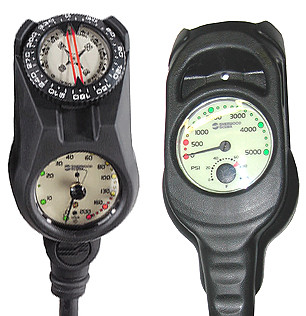The image features two black plastic pressure gauges set against a featureless white background. The gauges are placed side by side, with the left gauge displaying two dials, one above the other, and the right gauge presenting a single dial.

The left gauge's bottom dial is a pressure gauge, marked from 0 to 500 psi in increments of 10, 20, 30, 40, 60, etc. The dial has a white face, black markings, and a black pointer. Above the pressure gauge on the left is a compass, which shows cardinal directions (north, south, east, west) and angles in increments of 0, 60, 90, 120, etc., encircling the compass dial.

The right gauge mirrors the pressure gauge on the left, featuring a single dial marked from 0 to 500 psi. This gauge also has a white face with black markings and a black pointer. Additional red and green markings delineate pressure ranges; red represents psi from 0 to 500, while green indicates higher pressure values.

In summary, the image depicts two black plastic instruments designed to measure pressure, set against a stark white background. The left instrument includes both a pressure gauge and a compass, while the right instrument features only a pressure gauge.